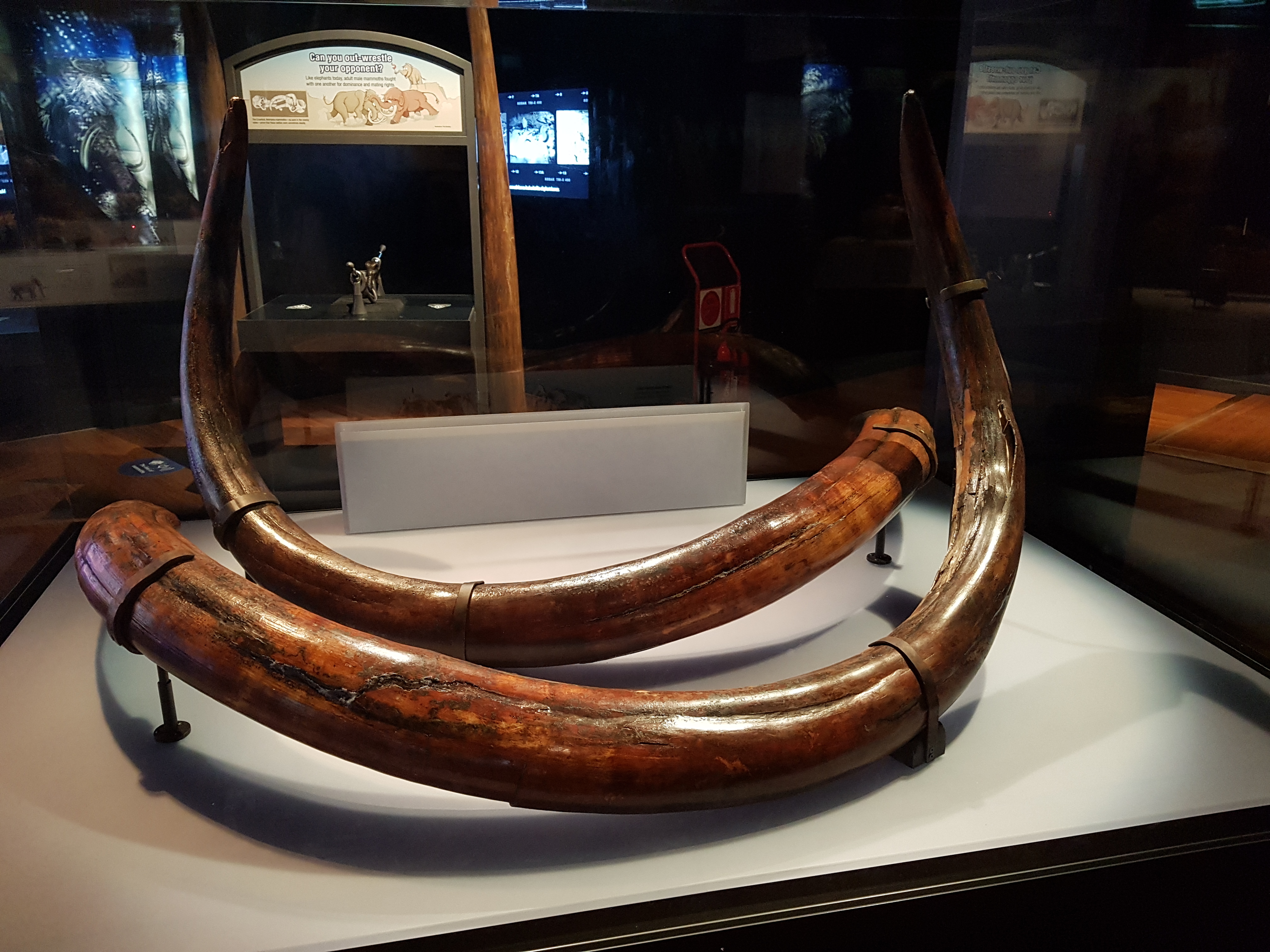The photograph captures what appears to be a polished and preserved display of curved, aged elephant tusks, rather than longhorn horns, secured on a white-colored base with metal supports. The tusks have been meticulously treated with preservatives, giving them a shiny, bronzed appearance. A reversed placard, possibly describing the tusks, is visible through the reflection on a protective glass case covering the exhibit. In the background, the setting resembles a museum or interactive exhibit space, featuring a dimly lit area with various displays. One notable display includes a sign that reads, "Can you out-wrestle your opponent?" accompanied by cartoon depictions of wrestling animals, including elephants, reinforcing the museum-like atmosphere.